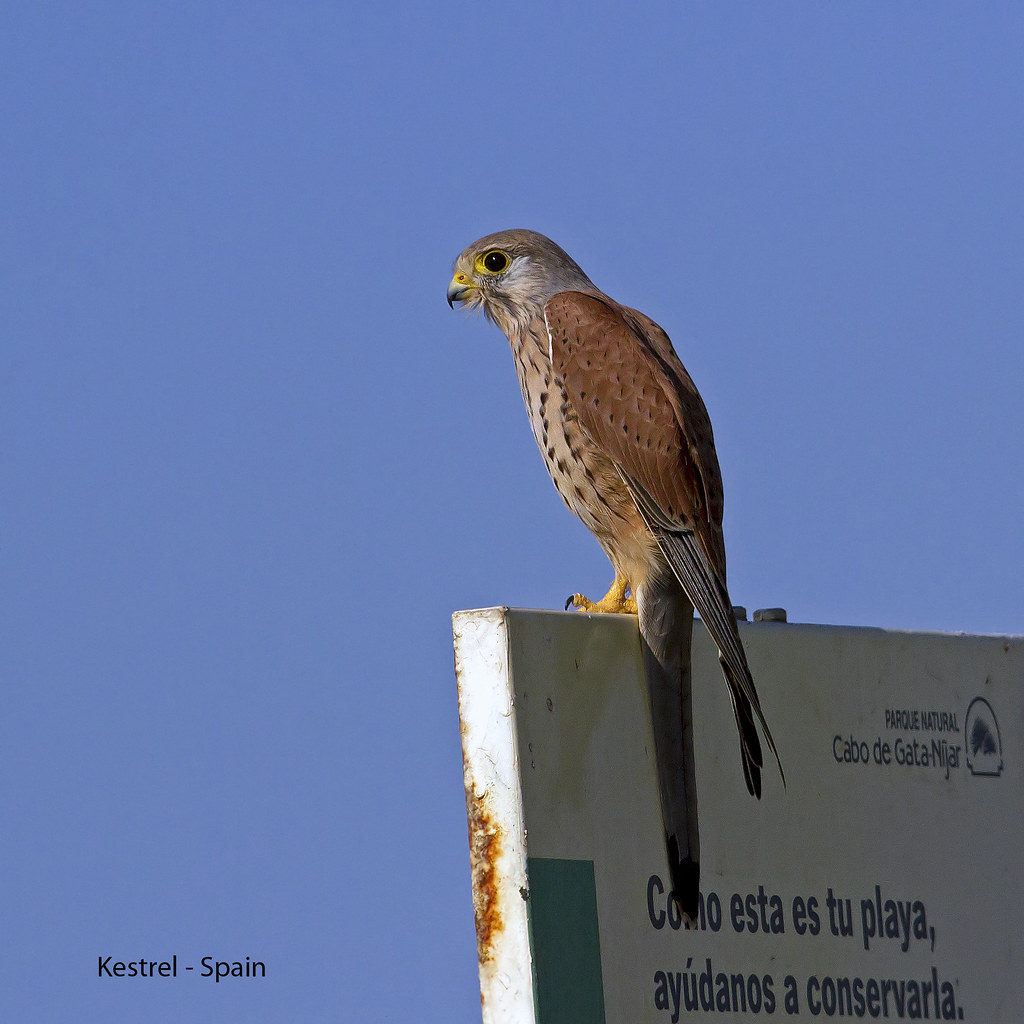This image depicts a hawk perched atop an old, rusted, white sign against the backdrop of a clear blue sky in Kestrel, Spain. The hawk is characterized by a grayish-brown head, yellow circular eyes, and a very short, hooked black beak. Its body features a light tan color speckled with black on the front, with darker brown wings adorned with dotted blacks on the feather tips. The bird also sports yellow feet equipped with sharp black talons. The sign, written in blue Spanish lettering, conveys the message: "Como esta es tu playa. Ayúdenos a conservar." Additionally, it bears the logo and name of the Parque Natural Cabo de Gata-Níjar. This sign aims to remind the public to help preserve the natural beauty of the area.